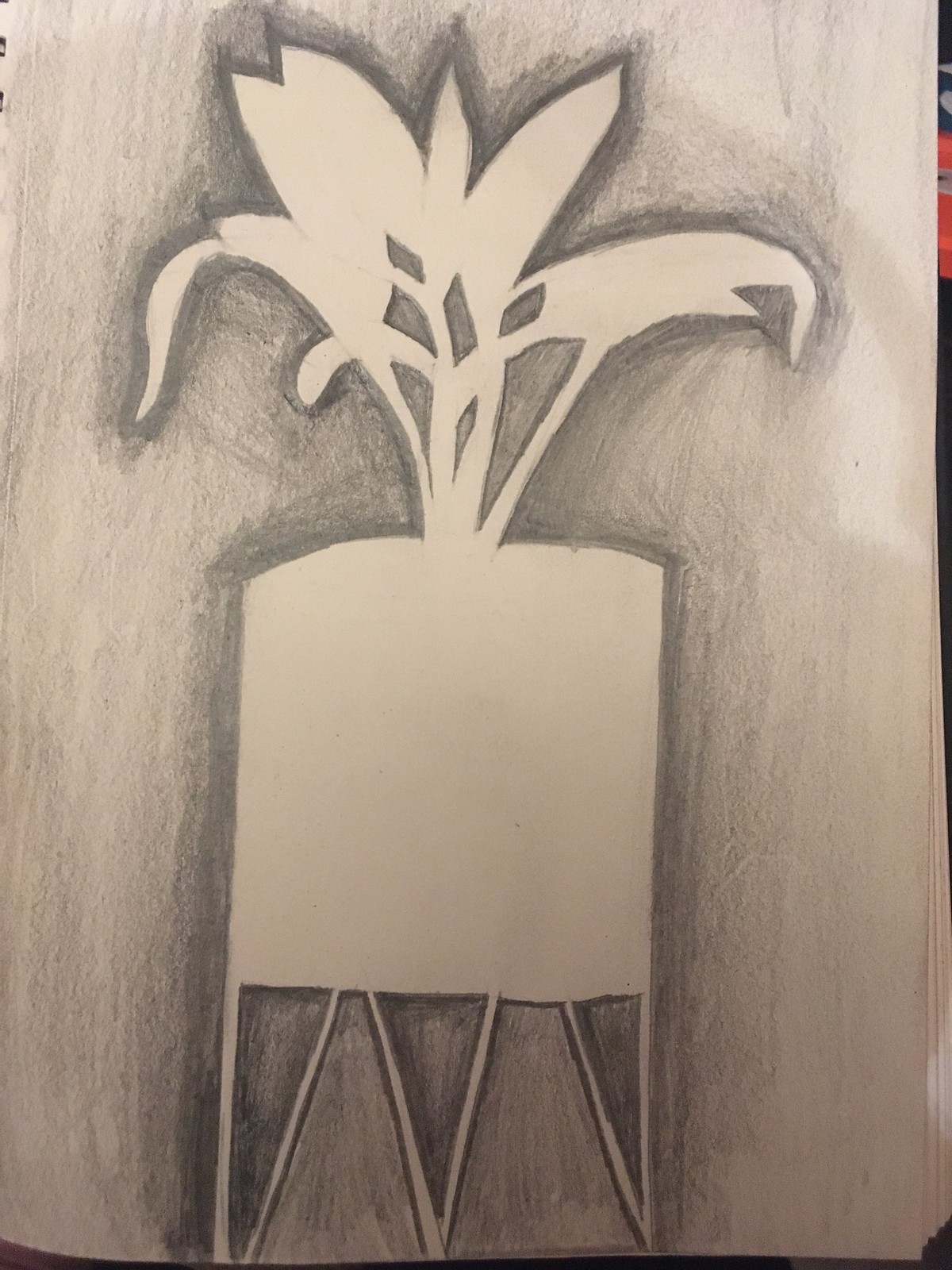This vertical graphite pencil sketch captures a striking image of a tank, supported by triangular, silhouette-shaped braces. The tank itself features a rounded, dome-like upper section and a spherical bottom, while its overall structure appears square from the midsection upwards. Emerging from the top of the tank, a plant grows in silhouette, adding an organic element to the otherwise industrial subject. Heavier shading around the tank, supports, and plant accentuates their forms against the white paper background. The composition lacks any identifying marks such as a date or artist's name, and appears to be drawn on a sheet from a spiral-bound artist's notebook.